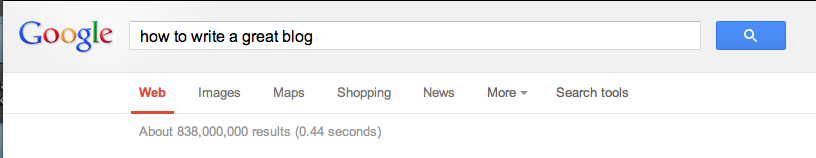This image captures a partial screenshot of a Google search result page. The image is framed with a distinct black border, thicker on the left side where it has a bluish hue intermingled, and thinner on the top edge. At the top of the screenshot, there is a long, horizontal rectangular box featuring the iconic Google logo composed of blue, red, yellow, and green letters. 

To the right of the logo, there is a search bar with a white background and black text where the query "how to write a gray block" is entered. Adjacent to this input box is a blue rectangular button with a white magnifying glass icon, indicating the search function.

Below the search bar, there are several navigation options displayed on a white background. The section shows tabs labeled "Web," "Images," "Maps," "Shopping," "News," "More," and "Search tools." The "Web" tab is highlighted in red, signifying it is the active tab. "More" includes a dropdown arrow, suggesting additional options.

Further down, a thin gray border precedes a line of text in gray font that reads, "About 838 million results (0.44 seconds)," indicating the search result count and the time taken to retrieve it. The image captures only a portion of the screen and focuses primarily on the search interface and statistical information related to the query.